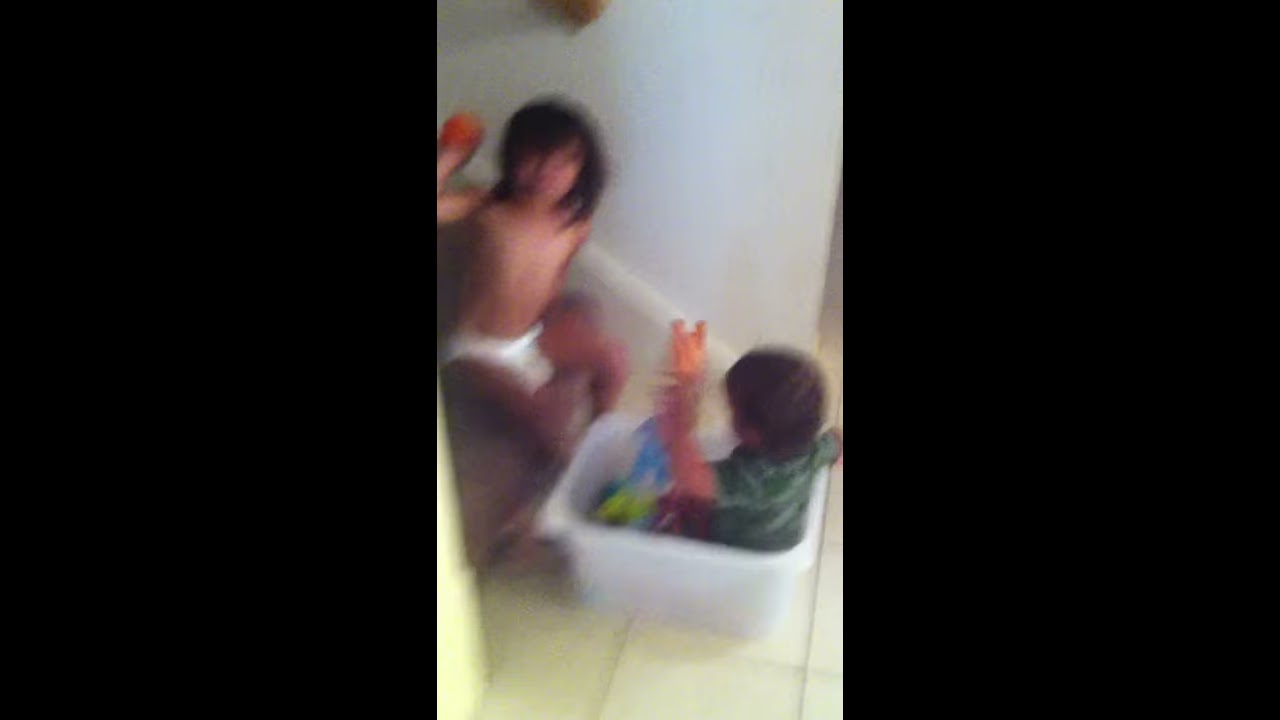In this low-quality, blurry photo, the setting is a bathroom with off-white tiled floors and plain white walls. The image captures a candid moment between two young children, one around four years old and the other about two. The older child, wearing only a diaper, stands poised to throw a ball at the younger child. The toddler, dressed in a dark green shirt, sits in a white plastic tub, holding an orange bunny rabbit toy aloft as if in self-defense. Additional toys, including a blue and green bunny, are also visible in the tub. A splash of color is provided by a yellow towel in the bottom left corner. The scene evokes a playful and slightly mischievous atmosphere, frozen in a moment of sibling interaction.